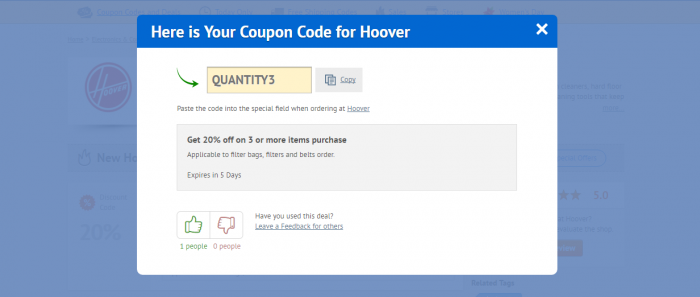This screenshot features a promotional pop-up for Hoover. The prominent red Hoover logo is visible in the background, while the pop-up itself has a blue header. In white text, the header reads: "Here is your coupon code for Hoover." Below, a green arrow points towards the message "Quantity 3," suggesting an option to copy a coupon code. Additional instructions in the pop-up advise users to "paste the code when you're ordering at Hoover." At the bottom, a grey box details an offer: "Get 12% off on three or more purchases," which expires in five days. The interface includes a green thumbs-up icon and a red thumbs-down icon for user feedback, and an 'X' at the top right corner for closing the pop-up. Faintly visible in the background are stars, adding a subtle decorative touch.